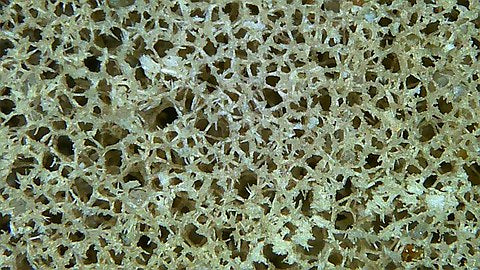The image is a highly detailed close-up photograph, likely captured in a landscape orientation, showcasing a complex, jumbled structure reminiscent of a sponge or plant matter. The dominant surface is yellow with a resin-like quality, interspersed with numerous holes and white spots. The structure has a crisscross, knitted pattern, and it bears a striking resemblance to either a sponge's porous texture or a plant's dense, bramble-like formation. The jumbled up appearance has a green hue that could resemble green crystal, giving it an underwater or biological feel. The background visible through the holes appears black, enhancing the contrast and adding depth to the image’s intricate details.